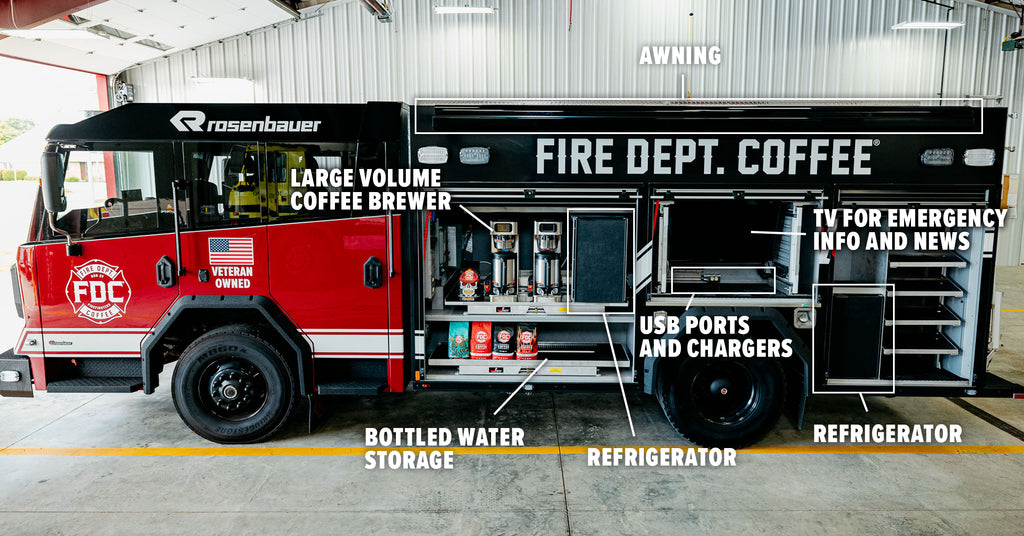The image depicts a red and black fire truck that has been transformed into a mobile coffee stand by Fire Department Coffee, a veteran-owned company. The truck is inside a large garage or warehouse and prominently displays the brand name "Fire Dept Coffee" underneath an American flag. Various components of the truck are clearly labeled with arrows indicating their locations, including a large-volume coffee brewer, bottled water storage, a refrigerator, USB ports and chargers, and a TV for emergency information and news. There's also a second, larger refrigerator in a different section and several shelving units. An awning, which provides shade when extended, is also referenced. The truck bears the brand Rosenbauer, and no people are depicted in the image.